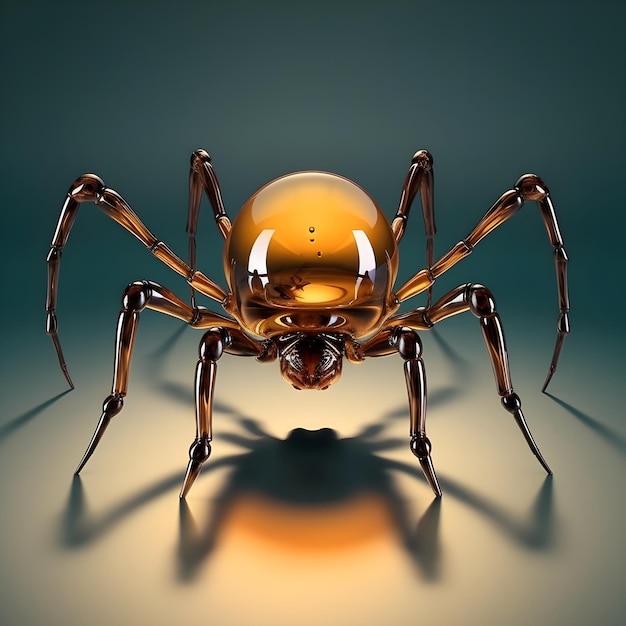The image seems to depict a digitally created or AI-generated spider, resembling a glass sculpture. The spider is predominantly brown with a shiny, translucent appearance that transitions from dark brown to black and lighter brown hues, giving it an artistic and cartoony vibe. Its large, round abdomen, reminiscent of amber or gold-colored glass, features intricate details such as air bubbles and a darker brown swirl in the center. The head is smaller and less defined, with the segmented legs all touching the ground. Beneath the spider, there is a distinctive blue and orange shadow. The spider stands against a gradient background that transitions from soft yellow at the bottom to dark teal at the top, enhancing the impression of depth and artistic flair.